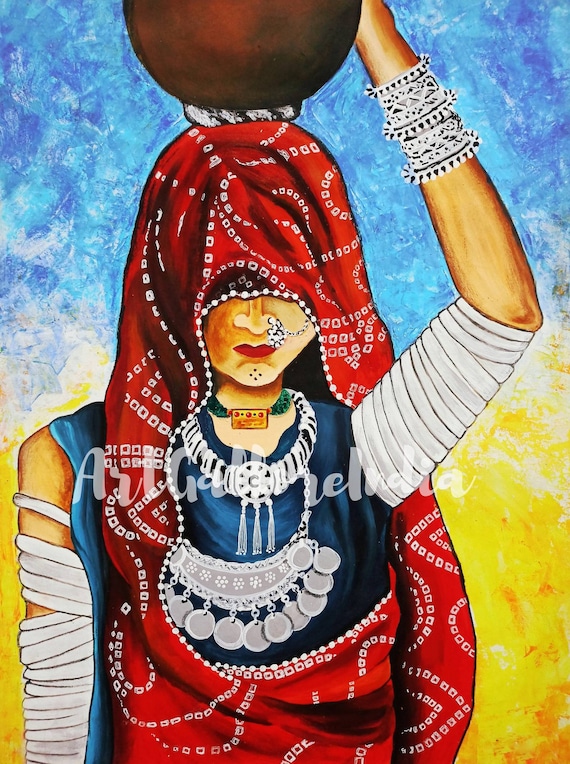The painting depicts a solemn young woman with light brown skin, dressed in a traditional outfit. She wears a red headscarf adorned with white beads that wraps around her head and drapes over her shoulders, obscuring her arms. Her blue and red tunic is sleeveless, revealing her biceps, which are wrapped with white cord reminiscent of mummy bandages. Her left arm is raised, holding a dark brown pot decorated with black and white patterns, balanced on her head. Silver bangle bracelets adorn her wrist. 

Her facial features include a nose ring that extends toward her eye, red lipstick, and a downward gaze, contributing to her solemn appearance. She wears a green choker with a golden plate, along with additional necklaces—one white and one silver with small bangles hanging. The background features blended tones of yellow at the bottom and varying shades of blue at the top. Across the center of the image, there is a faded white print that partially reads "Art G-A...India," suggesting a possible poster or artistic label.